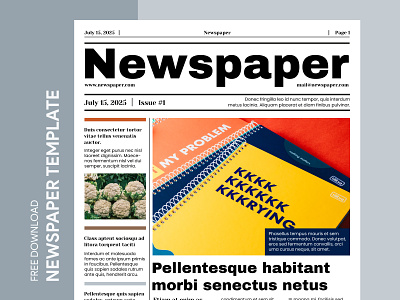The image portrays a newspaper page against a dual-tone gray background, with the left side being dark gray and the right side light gray, divided approximately in a one-third to two-thirds ratio. The newspaper itself bears the title "Newspaper" in bold black letters at the top. Directly beneath the title, the date is listed as July 15, 2025, followed by the issue number, which is "Issue Number One". The newspaper contains a central color picture displaying two spiral-bound notebooks - a yellow one with several “K” letters on its cover, resting atop a blue one, set against a red background. To the left side of the newspaper page, there are vertically aligned words stating "Free download newspaper template" in white print. Additionally, below the main title, there is a headline written in a foreign script, "Palintiske Habitant Morbi Sanctus Nectus". On the right-hand side, beneath the headline, there is a small column with an accompanying picture and article text.